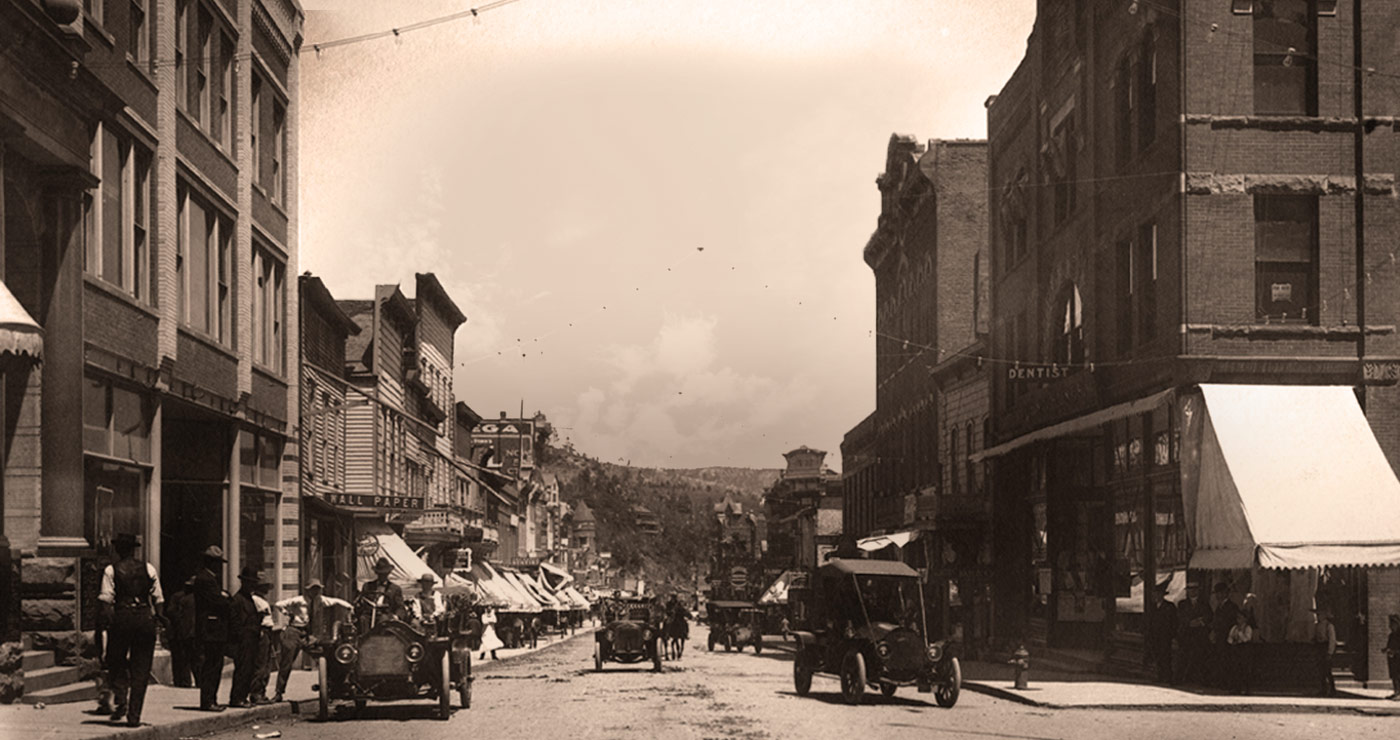This vintage photo, likely from the 1920s, portrays a busy street scene in a developing small town in the USA. Taken in a brownish black-and-white style, the image captures a moment in time with a nostalgic hue, perhaps due to its age. The street stretches ahead, lined with storefronts on both sides that likely have apartments above them. Early cars, reminiscent of Model T types, drive along the street, and several pedestrians mill about, dressed in typical 1920s-1930s clothing. In the background, the hazy sky hints at clouds, with distant hillsides visible along the horizon. The left side of the street is bustling with people walking on the sidewalk, while on the right side, stores and a fire hydrant are noticeable. The overall scene illustrates everyday life in the developing city, combining the elements of commerce, travel, and community interaction from that era.